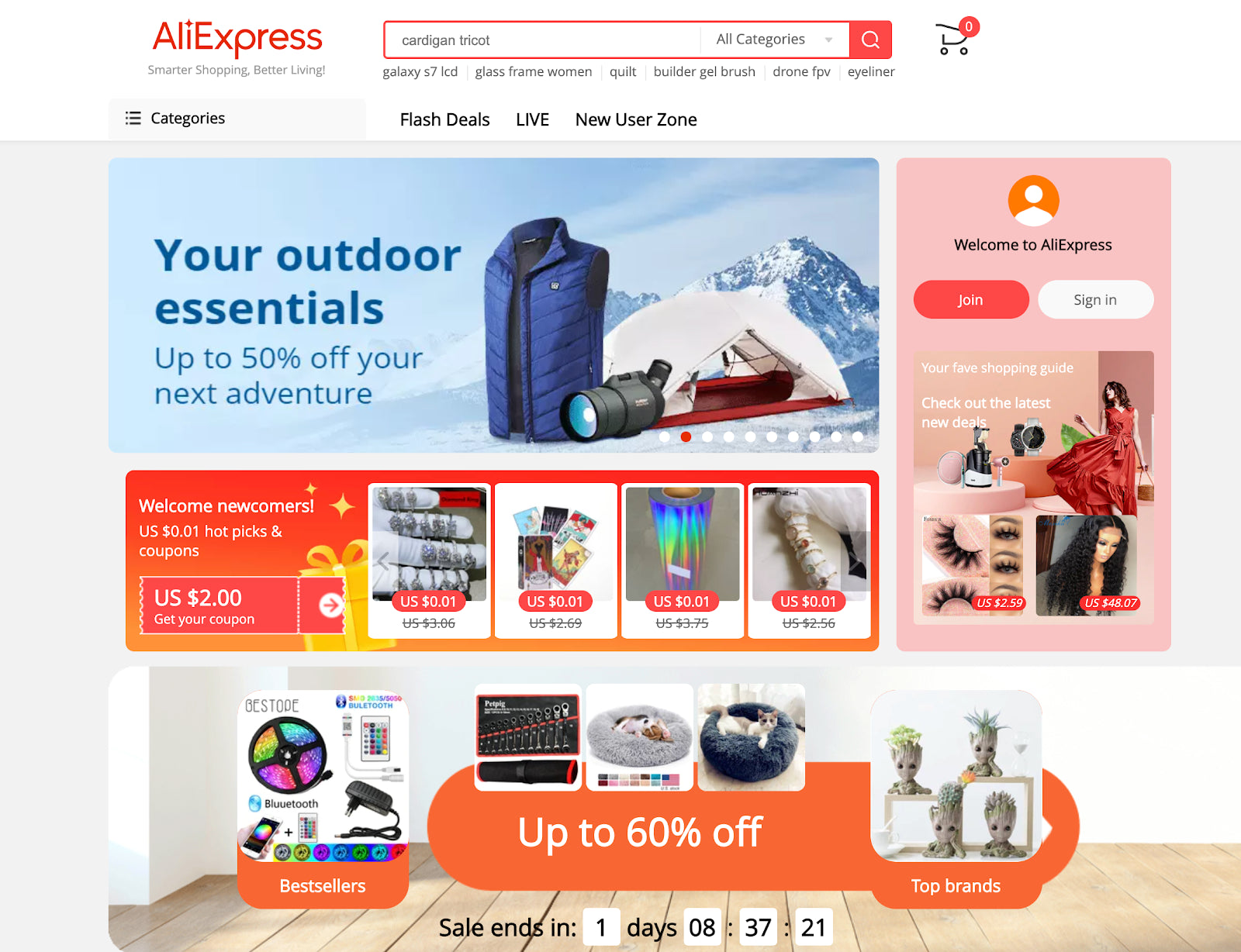The image showcases a vibrant AliExpress homepage filled with various promotional banners and offers targeting both new and existing users. In the forefront, a banner highlights “Outdoor Essentials” with discounts up to 50% for your next adventure, featuring a vivid illustration of a telescope, a tent, and majestic mountains in the background. 

Below this, another section promotes “Flash Deals” and “Live New Users,” introducing newcomers with enticing offers such as “U.S. One Cent Hot Picks and Coupons” and “U.S. Two Dollar Coupons.” An image of a girl in a dress, alongside items like eyelashes, a camera, and a wig, welcomes newcomers to join and sign in.

Further down, a colorful assortment of items grabs attention, showcasing bestsellers: a colorful wheel, a black plug, a keyboard, a gray and blue pet bed, and an adorable clay Groot figure from "Guardians of the Galaxy" with plants sprouting from it. 

The bottom section advertises “Top Brands Up to 60% Off” with a countdown timer indicating the sale ends in one day, eight hours, thirty-seven minutes, and twenty-one seconds, urging users to make the most of the limited-time offers.